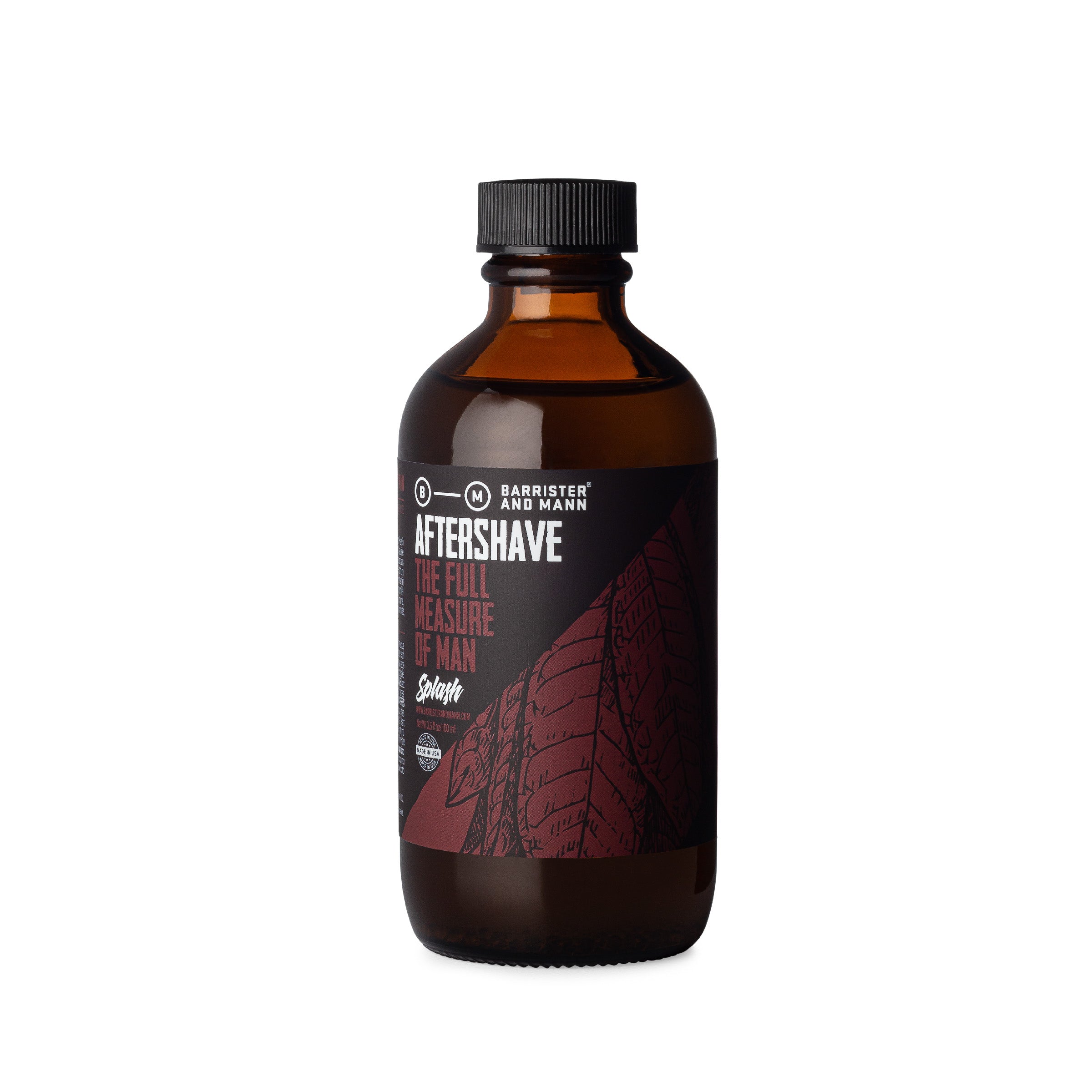The image showcases a small, dark amber glass bottle of aftershave with a simple yet elegant design. The bottle features a black lid and is nearly filled with liquid. Prominently displayed on the front is a dark black label with various texts and images. The label reads "Barrister and Mann" at the top, followed by "Aftershave" in bold white text. Below that, in deep red text, it says "The Full Measure of Man," and further down in an almost cursive, italic white font, is the word "Splash." Below this are two more lines of text that are too small to decipher. To the bottom right of the label, on a triangular shape, is an intricate illustration of leaves, appearing to be veins and lines in a black-red gradient. Additionally, there is a small circular logo featuring letters that appear to be "B" and "M," though it is difficult to make out entirely. This detailed depiction captures the refined and sophisticated appearance of the aftershave bottle, highlighting its luxurious and crafted aesthetic.